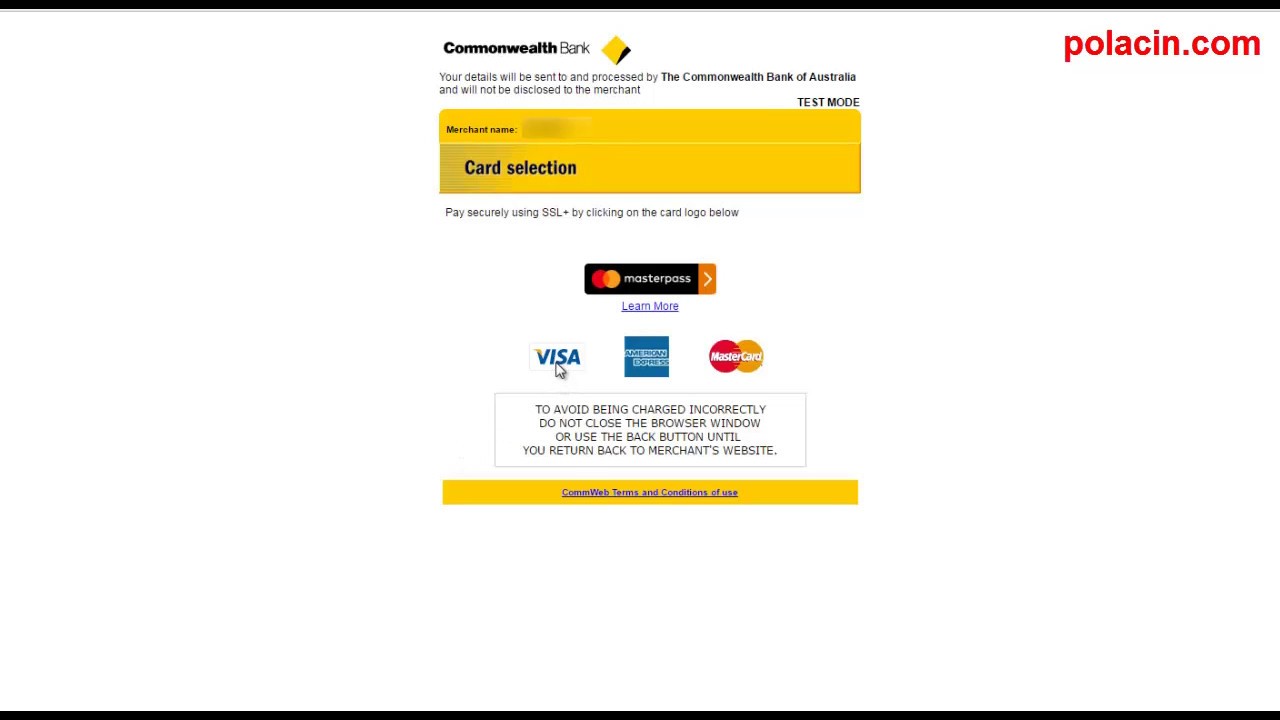*Screenshot Description: Commonwealth Bank Payment Portal*

The screenshot appears to be taken from either a smartphone or a website, primarily displaying a payment portal. 

At the top right of the image, the text "polacin.com" is noticeable in red, indicating the domain of the website. This text stands out against the stark white background, flanked by two thin black horizontal borders.

Below these details, the logo of Commonwealth Bank is prominently featured. The logo, a distinctive diamond shape, is primarily a golden yellow with a black segment on its left side - a design consistent with the bank's branding colors.

Underneath the logo, informative text states: "Your details will be sent to and processed by the Commonwealth Bank of Australia and will not be disclosed to the merchant." The name of the bank is bolded for emphasis.

Below this information, the text "TEST MODE" is displayed, followed by “Merchant,” with two bars in golden yellow beneath it, potentially for user input, though the specific merchant name is blanked out in this screenshot.

Further down, the section titled "Card Selection" provides instructions, stating: "Pay securely using SSL by clicking on the card logo below." This section includes icons for various payment methods: MasterPass, Visa, American Express, and MasterCard.

An important notice at the bottom cautions users: "To avoid being charged incorrectly, do not close the browser window or use the back button until you return to the bank."